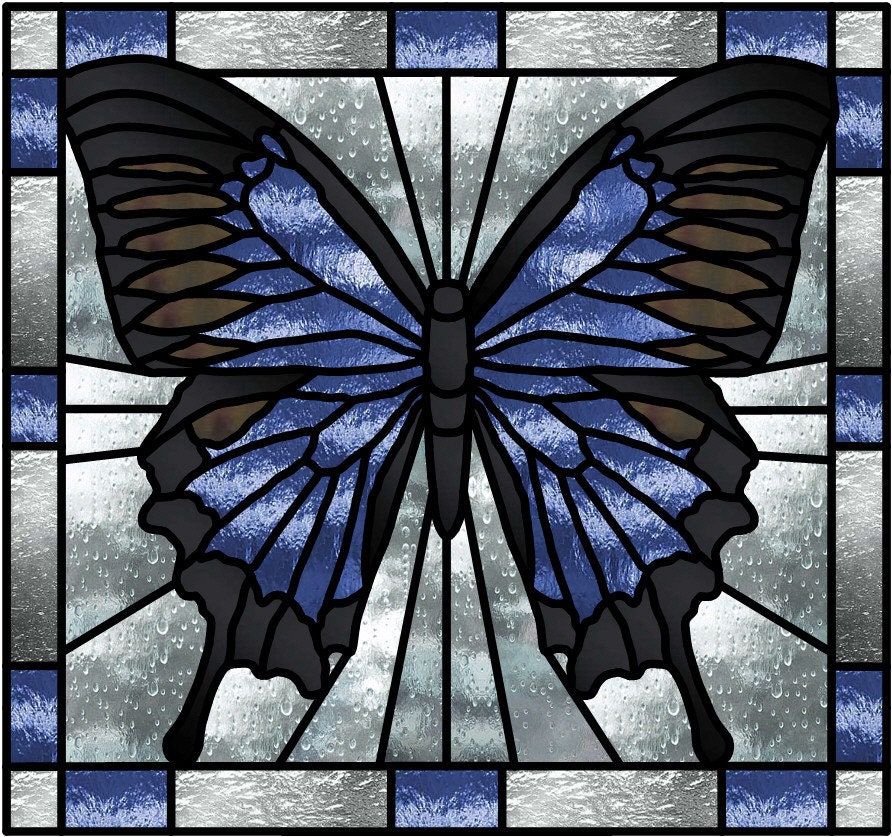This image captures a stunning stained glass window designed in the shape of a butterfly. The window is completely square, with the butterfly dominating the central portion. The butterfly itself is primarily blue, with its wingtips adorned in shades of brown and black. The edges of the butterfly’s wings are outlined in black, with the inner sections displaying a mix of blue and brown hues. The butterfly's body is also black, blending seamlessly with the wings.

The window features a decorative border comprised of alternating blue and clear rectangles in a consistent pattern surrounding the butterfly. The frame around the stained glass appears silver in contrast to the vibrant colors within. The stained glass has a captivating detail where water droplets are visible on the outer side, suggesting a recent rain, adding to the overall allure of the piece. The intricate design and rich colors imply that it would be exceptionally beautiful under full light.